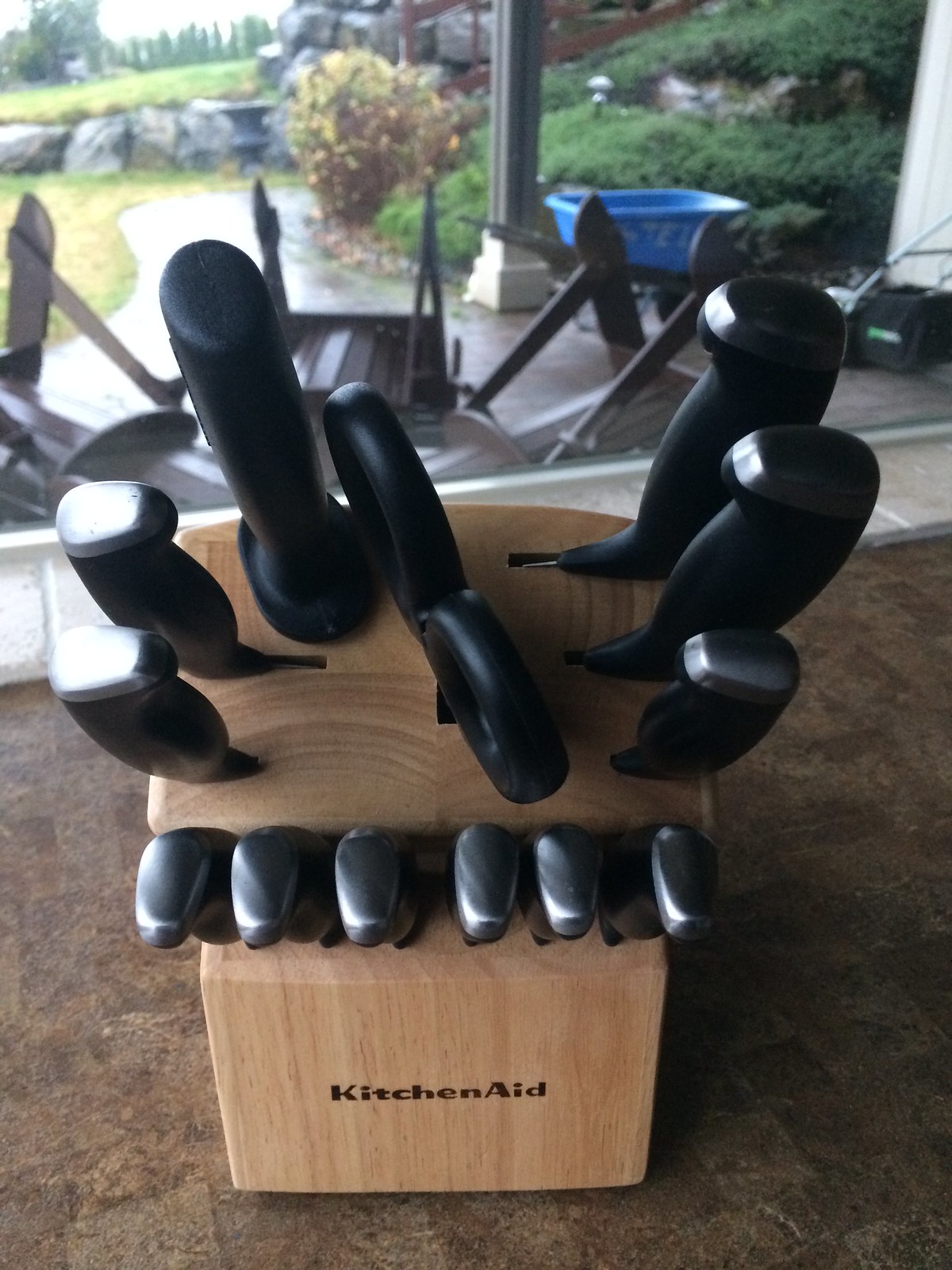The image showcases a detailed and focused view of a wooden KitchenAid knife block, prominently displaying the brand name "KitchenAid" at the lower front. The knife block, resting on a brown, laminate or marble-like countertop, features an array of black-handled knives marked with white lines. The arrangement includes six small knives at the bottom, a pair of scissors positioned centrally, flanked by three knives on either side with varying sizes—from large to medium to small. In the outdoor background seen through a window or open area, we observe an upside-down arrangement of tables and chairs, a wheelbarrow with a blue barrel, a possible lawnmower on a concrete pathway, a pillar, and a gradient of greenery and plants leading up to a rocky wall. This scene, characterized by lush grass and distant trees, suggests a yard space, enhancing the kitchen's open and connected ambiance to the outdoors.